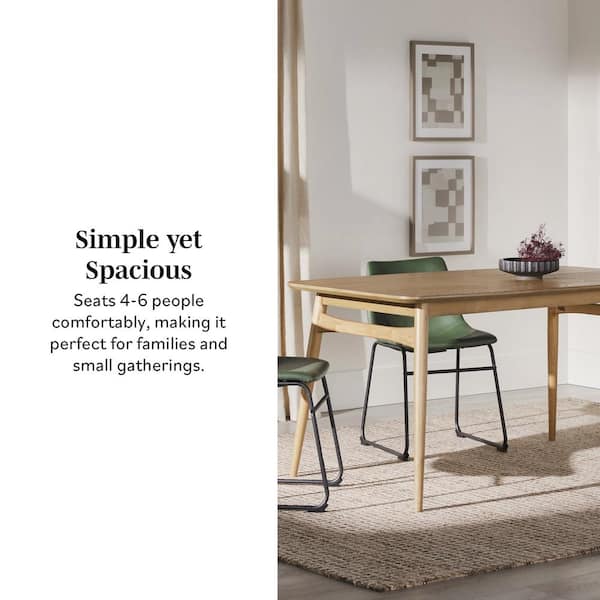This advertisement features a modern dining table set in a brightly lit, sunlit room. The table, made of beige wood with sleek, contemporary lines, sits on a light cream-colored floor, atop a dense, beige woven rug. Flanked by two olive-green chairs with thin, wiry legs, the setup exudes a minimalist charm. A gray bowl with a small plant adds a touch of nature to the table's surface. Behind the table, a white wall is adorned with two abstract, brownish-cream paintings, framed in dark gray-beige. On the left side of the image, bold text reads, “Simple yet spacious,” highlighting that the table seats four to six people comfortably, making it perfect for families and small gatherings. This detailed visualization combines all elements to showcase a functional yet elegant dining space.